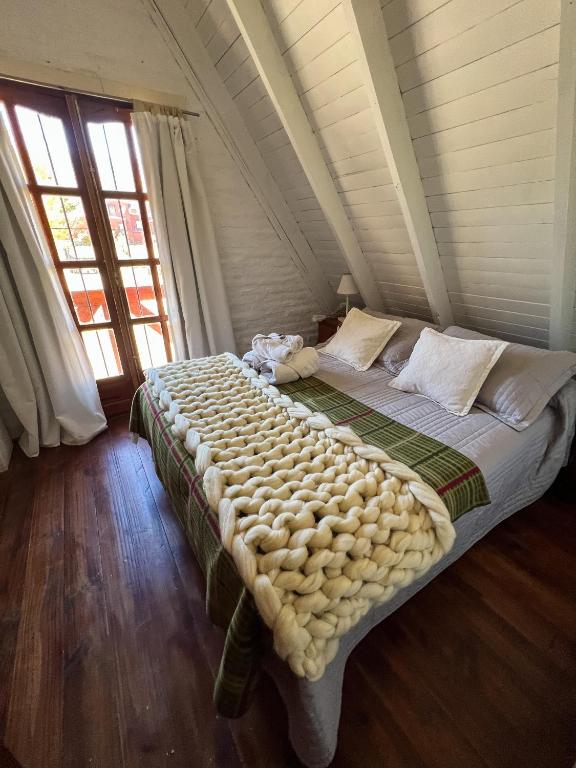This image features a spacious, country-style attic bedroom, characterized by its distinct architectural features. The right side of the room showcases an angled ceiling with visible wooden slats, painted white, contributing to the room's rustic charm. The finished space includes dark brown, large plank hardwood floors that enhance its cozy aesthetic.

A king-sized bed is positioned against the angled wall, adorned with a layered arrangement of bedding. This includes a green plaid blanket at the edge, a light gray comforter, and coordinated beige and gray pillows, with white accent pillows adding a touch of brightness. Draped over the bed is a chunky, beige knitted throw with a pronounced cable pattern, resembling oversized yarn, adding a textural and cozy element to the decor.

On the left side of the room, large wooden French doors with square glass panels open out to a balcony, allowing abundant natural light to flood the space. The doors are framed by white curtains held open by a curtain rod above. A brown nightstand with a lamp stands near the bed, adding functionality and charm to this serene attic retreat.